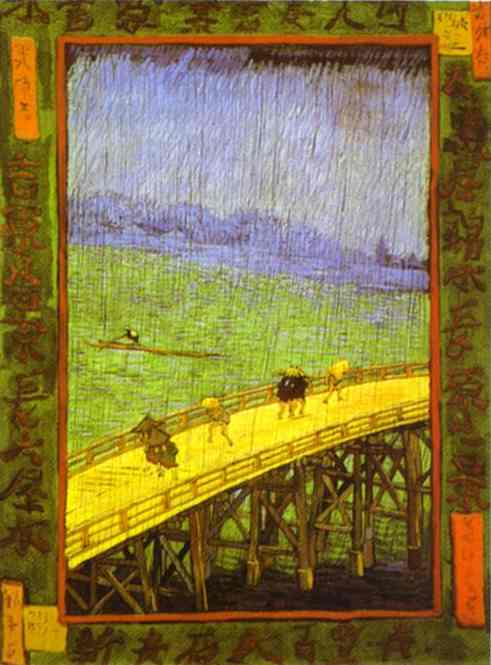The painting, characterized by its primitive lines and textured surface that suggests it might be painted on wood, showcases a detailed old-world scene with a slight blur. At the center is a yellow bridge elevated on wooden stilts, crossing over green water. Six figures, dressed in traditional clothing and wearing wide-brimmed, conical hats, traverse the bridge. Two groups of two walk in opposite directions, each followed by a solitary figure. Beneath the bridge, a long, narrow boat navigates the water. In the distance, there are mountains and trees, set against a pale whitish-blue sky. The artwork is framed by a smudgy olive-green border adorned with black Asian characters, which may suggest a Japanese or Chinese influence. The entire scene, with its cartoonish or older Asian style, evokes a serene, nostalgic atmosphere.